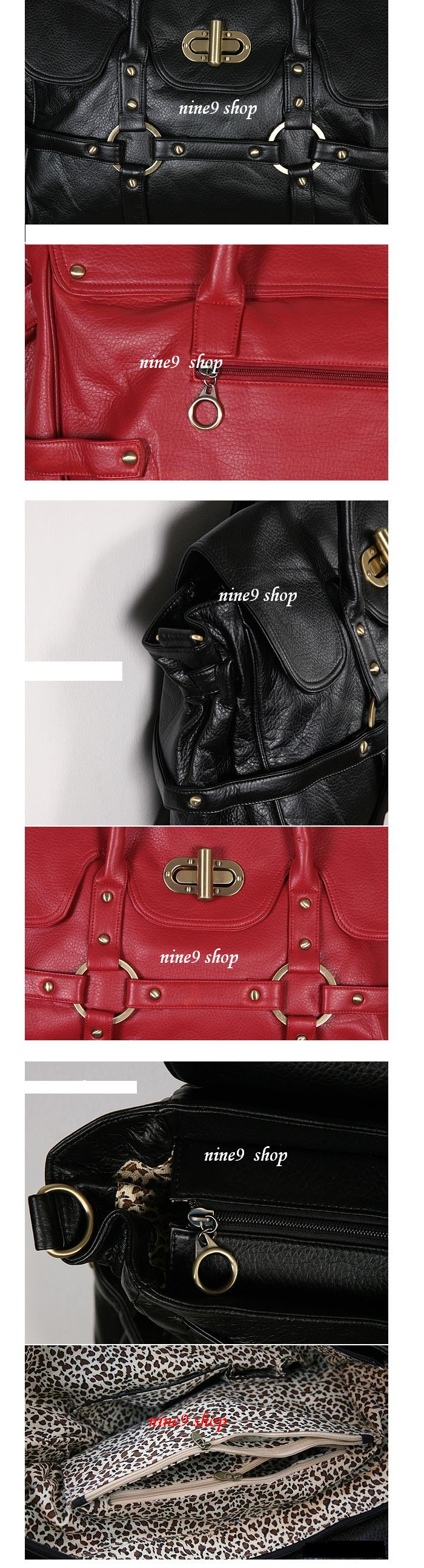This image is a vertical collage of six detailed product photos, tailored for a website listing or poster. Each photo features a handbag from the Nine-Nine Shop, showcasing different colors and angles of the same style bag. The sequence starts with a black leather handbag adorned with gold hardware and a signature buckle. Below it is a red leather handbag with silver hardware, highlighting its zipper area. The third image circles back to the black handbag, captured from a side angle to reveal its strap and flap closure. Next is another angle of the red handbag, centering on its golden clasp and straps. The fifth photo returns to the black handbag, focusing on its zipper with a prominent metal ring pull. The final image presents the interior of the bags, displaying a black and white leopard print lining, complete with inside compartments and pockets. Each bag is positioned against a plain white background, with a watermark in a small, white italic serif font reading 'Nine-9 Shop'. Despite the heavy use of flash, the photos provide detailed views of the handbags’ materials and craftsmanship.